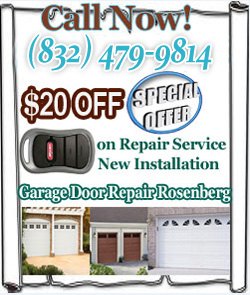### Detailed Caption for Image

The image is a screenshot of a section of a webpage, presented with a design mimicking an unrolled scroll. The background of the page is white, outlined in black, and features two black-outlined rolls on either side, giving the scroll appearance. The top and bottom edges of the page are irregular and uneven, contributing to the scroll effect.

At the bottom of the webpage, there are images of three different types of garage doors. From left to right:
1. The first is a cream-colored double garage door, or possibly two single doors, featuring four windows with brown trim.
2. The second is a pair of red single doors, each with two windows at the top.
3. The third is a white double garage door with four sets of partial windows that arch slightly in the middle.

At the top of the page, prominent red text reads "CALL NOW!" followed by a phone number in parentheses: (832) 479-9814, displayed in blue. Below this, there is a red banner outlined in white with the text "$20 OFF."

To the right of this banner is a blue circle with "SPECIAL OFFER" in white letters shaded in black.

Beneath these promotional texts is an image of a gray and black remote control with a red button, lying on its side. Green text nearby reads "ON REPAIR SERVICE, NEW INSTALLATION."

At the bottom of the page, there is also a heading in black text: "Garage Door Repair Rosenberg."

This comprehensive layout and detailed graphics promote garage door repair services, emphasizing special offers and contact information.